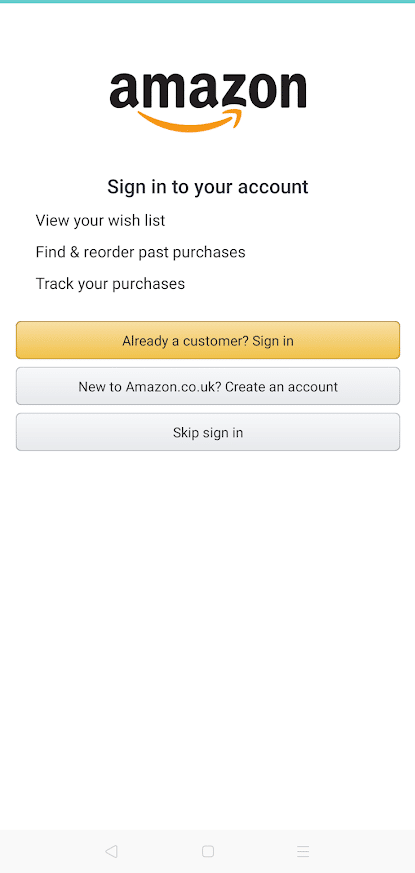The image depicts a login screen for an Amazon.co.uk account, prominently featuring the well-known Amazon branding and logo, which includes the distinctive orange arrow underneath the Amazon name. Below the branding, a prominent header reads "Sign in to your account" in a slightly larger font. This is followed by three options in a smaller font: "View your wish list," "Find and reorder past purchases," and "Track your purchases."

Under these options, there are three separate buttons for user actions. The first button, highlighted in yellow and set as the default choice, prompts existing customers to "Sign In." The second button offers new users the option to "Create an Account" if they don't already have one. The final button allows users to "Skip Sign In."

Overall, this image provides a clear and organized snapshot of the Amazon login interface, emphasizing the easy access to account management and shopping functionalities.